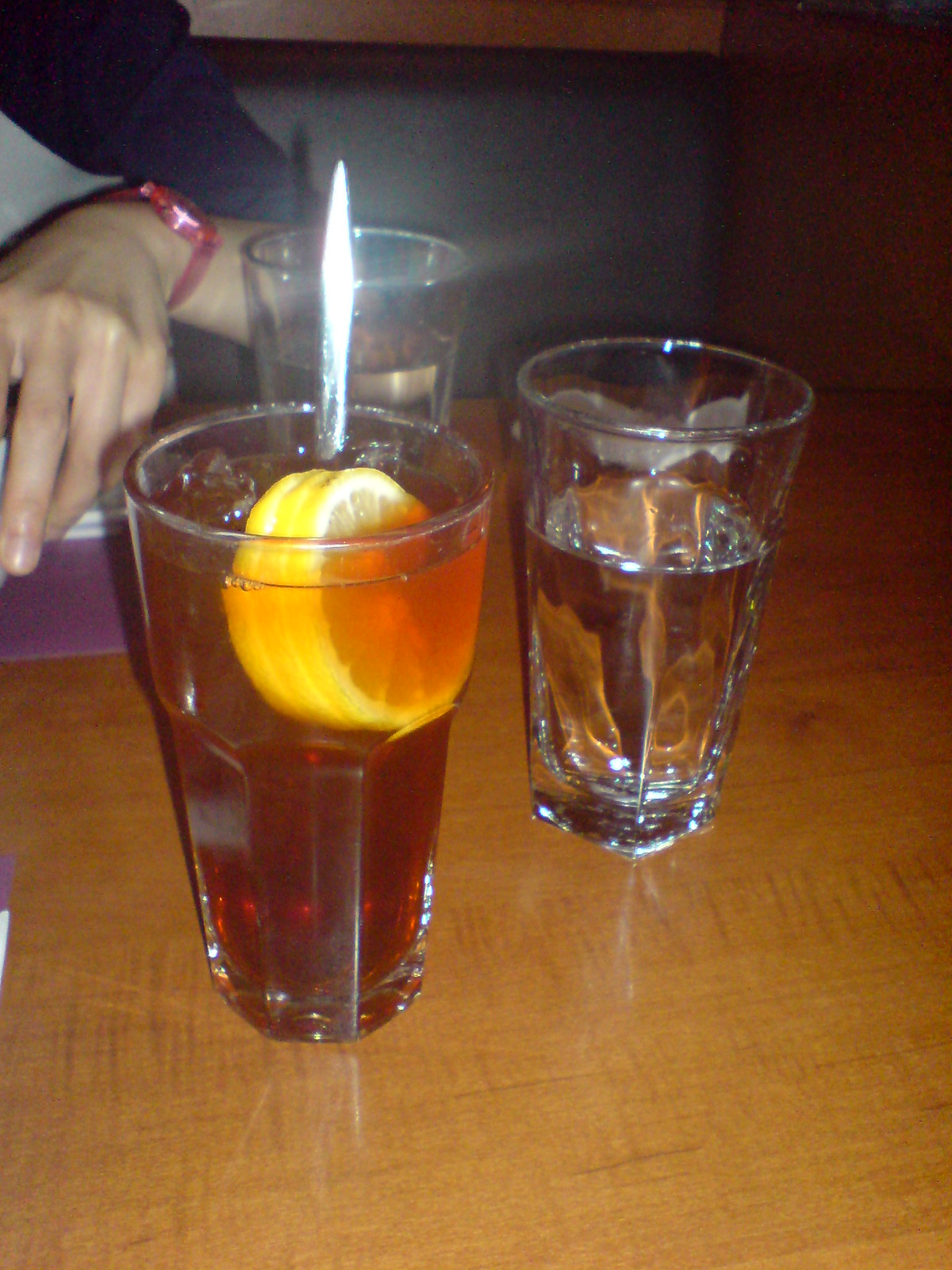The photograph captures a detailed and somewhat enigmatic scene featuring a tall, heavier style clear glass of iced tea on a shiny, wood grain synthetic surface. The glass contains three full, thin slices of lemon, numerous clear, crushed ice cubes, and a white straw or stirring spoon that catches the light in a way that almost gives it a fiery appearance. To the right of this glass, there is a smaller glass of water, filled about two-thirds of the way, and a similar glass is seen in the blurry background. Adding a human element, an individual—seemingly a woman—wearing a pinkish or red watch is partially visible; her left wrist extends into the frame, suggesting she is seated at the table. The background is dark and out of focus, drawing more attention to the iced tea, the lemon slices, the ice, and the intriguing white straw.